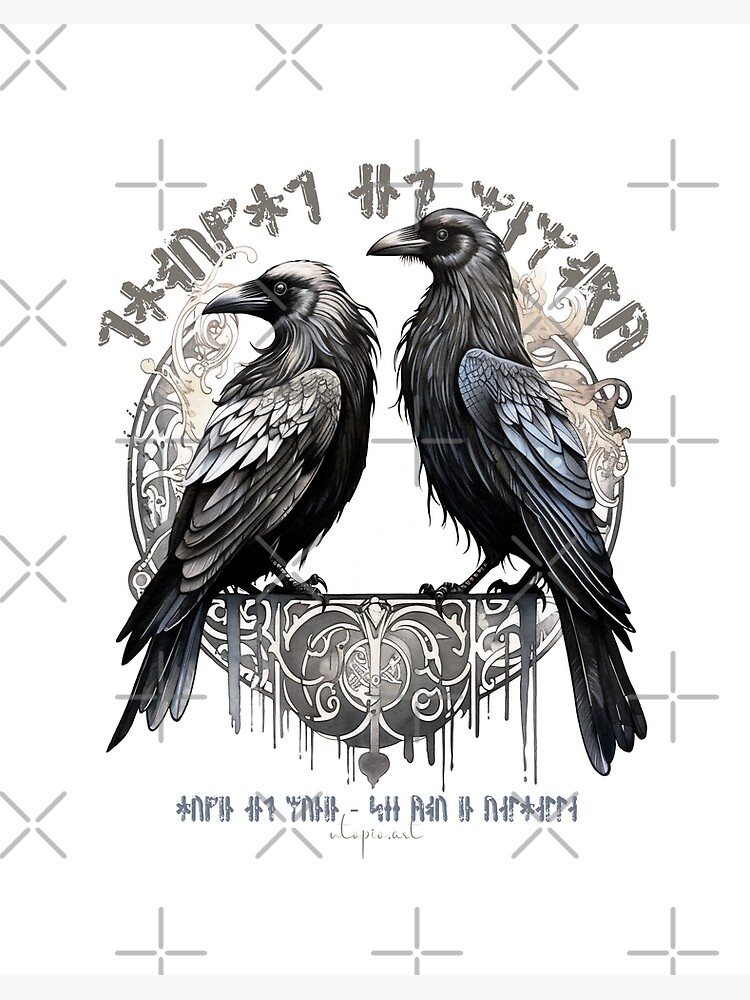The image is a detailed black and white drawing of two birds, likely crows or ravens, perched on an ornate, gray centerpiece with swirling patterns. The birds are identical in size but differ in feather highlights—one displays blueish tones while the other carries grayish hues. Both birds are positioned to face each other, yet their heads are turned to the left. Above and below the birds, there is text in what appears to be an Asian script, though it's not clearly legible. The white background is subtly detailed with faint Xs and crosses, adding an element of texture to the scene. The artwork is accented with gold and silver tones, contrasting with the predominantly black, white, and gray color scheme, making the image both intricate and visually striking.